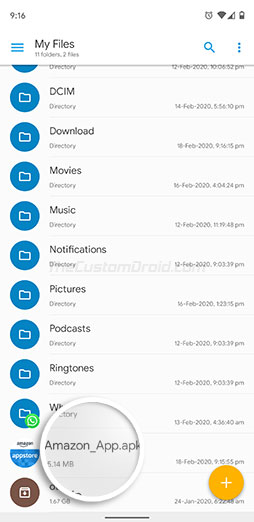A screenshot of a file directory viewed on a mobile device in vertical format is shown. The status bar at the top displays the time as 9:16 in the upper left corner, while the upper right corner shows a clock icon, indicators for cellular data, Wi-Fi signal, and a half-filled battery. Below the status bar, there is a section with three horizontal blue lines, accompanied by the text "My Files" and the status of "11 folders, 2 files." Positioned to the right are a magnifying glass icon for search functionality and a vertical ellipsis (three dots) for additional options.

The main content area is populated with profile-style blue circular icons, each featuring a white file folder symbol. These icons are labeled respectively: "DCIM directory," "Download directory," "Movies directory," "Music directory," "Notifications directory," "Pictures directory," "Podcast directory," and "Ringtones directory." A white circle magnifies part of this section, highlighting a file named "Amazon_app.APK" with the label "Amazon App Store" next to it. Additionally, a yellow circle with a white plus sign is visible on the right-hand side of the screenshot.